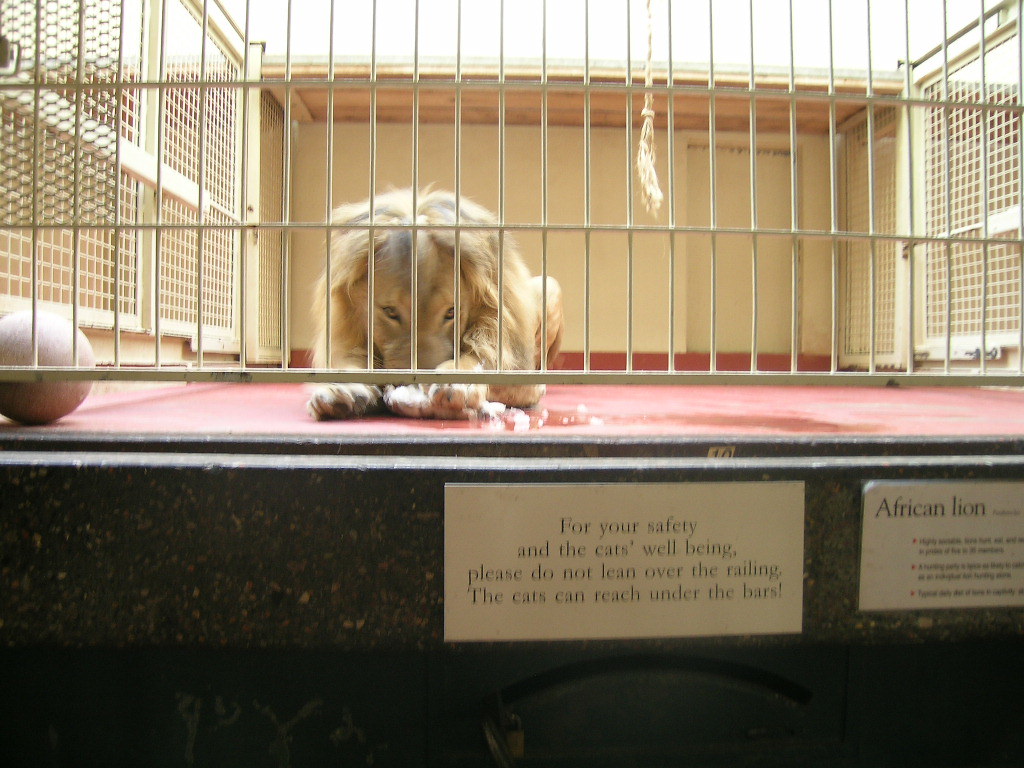This image captures a young male African lion enclosed in a well-lit cage, taking up the entirety of the frame. The lion, identifiable by its modest mane, is positioned centrally but slightly towards the left and is depicted lying down. The floor of the cage appears to be hard, likely concrete, with some noticeable wet spots. The lion is seemingly engaged in chewing something. A red play ball is visible in the left corner of the cage, along with a rope toy by the lion’s side. The photograph is a bit blurry, with the cage bars in focus while the lion remains slightly out of focus.

In the foreground, there are two prominent signs affixed to the cage platform. The left sign reads, "For your safety and the cat's well-being, please do not lean over the railing. The cats can reach under the bars." The right sign, partially cut off by the photo's frame, states "African lion" with additional smaller text beneath it that is too small to be legible. Both labels are rectangular, with a white background and black serif font, adding an informative constraint to the scene. The setting is bright, indicating the presence of natural light, possibly suggesting an outdoor zoo environment. The colors in the image include black, white, gray, tan, red, and yellow, contributing to the vibrant and naturalistic portrayal of the lion's habitat.